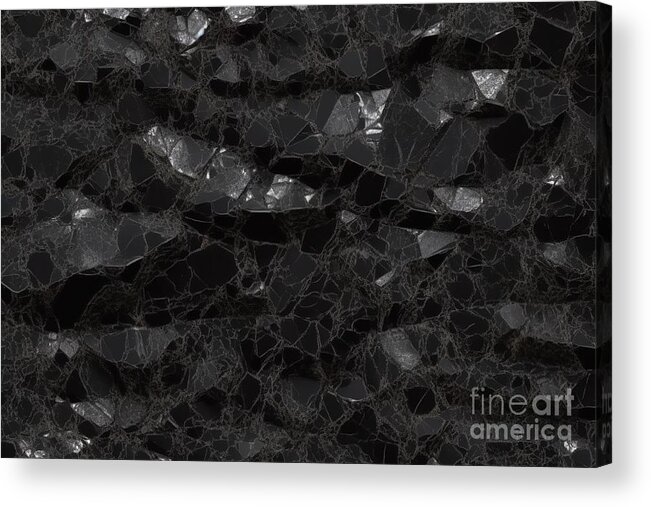The image features a stunning piece of abstract art resembling a mosaic, with a cracked-shatter effect that appears to be composed of different shades of black, grey, and white. Displayed on a canvas, the mosaic-like texture extends seamlessly to the sides, enhancing its 3D appearance. Dark black stones overlap and layer with lighter gray ones, some of which are adorned with white scratch marks. The entire piece exudes a metallic and shiny quality, with the patterns giving the impression of shards of charcoal or shattered glass. The fine cracks between stones add a sophisticated and intricate detail to the overall design. Positioned in the lower right corner is a watermark in bold, gray letters that reads "Fine Art America." The piece conveys a contemporary aesthetic, making it a suitable choice for modern interiors like kitchens or bathrooms.